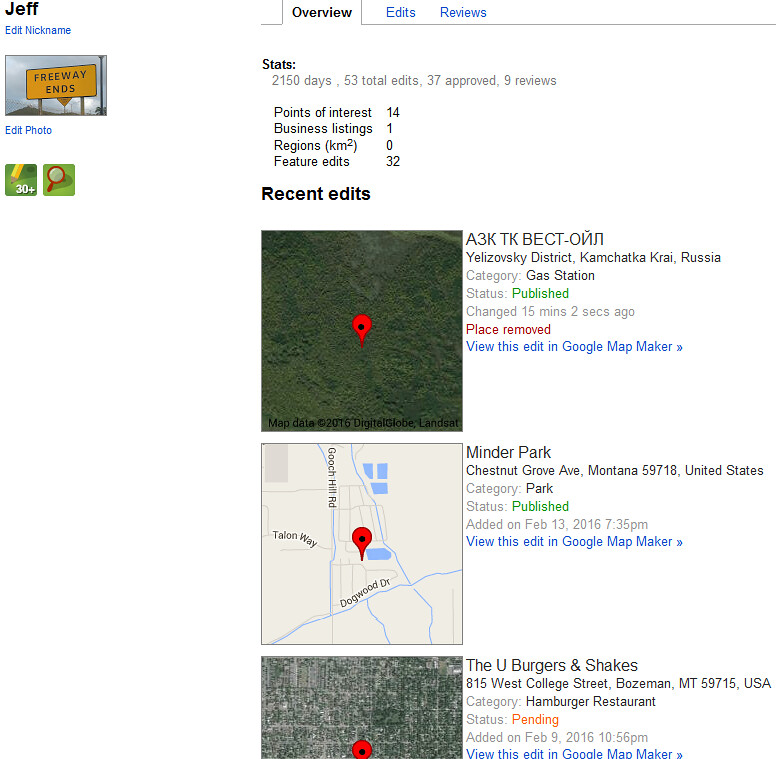This screenshot showcases a user's map overview page, prominently displaying their profile and editing statistics. In the upper left-hand corner, the user is identified as "Jeff" in black text, accompanied by a blue "edit nickname" link below. An icon signifying the end of a freeway, an "edit photo" option, a pencil marked "30+" and a magnifying glass symbol are located further down.

Dominating the center of the image are three tabs, with the "Overview" tab currently selected. This tab provides a summary of Jeff's contributions and activities. Below a "Stats" heading in black text, gray text indicates Jeff's statistics: 2,150 days of activity, 53 total edits, 37 of which have been approved, and 9 reviews. To the right, four detailed statistics are listed: 14 points of interest, 1 business listing, 0 regions, and 32 feature edits.

Further down, a "Recent Edits" section highlights Jeff's latest contributions, which include a landmark in Russia depicted as a forest with a red pin in the center. Another entry shows "Minder Park" located in Montana, also marked with a red pin, set in a suburban area. Additionally, an image of "U Burgers and Shakes" in Bozeman, Montana is shown with a top-down perspective of the map.

Adjacent to the "Overview" tab are the "Edit" and "Review" tabs, distinguished by their blue text.